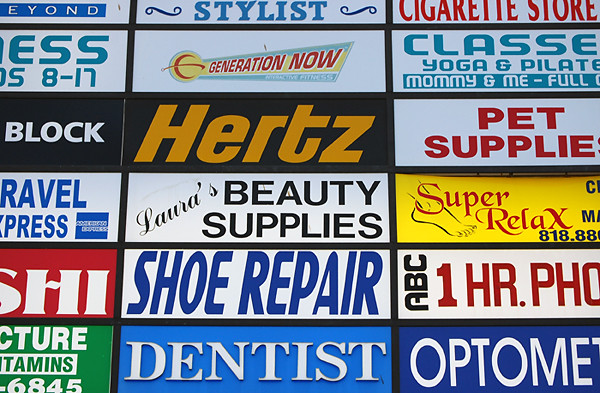This image captures a grid-aligned array of business signs, typical for a shopping or strip mall. The signage is organized into three vertical columns, each containing six rows, though the full visibility of signs varies. The central column is fully visible and prominently features signs for various businesses: at the top, a partially visible white sign with "Stylist" in blue, followed by a white sign with a sun and "Generation Now" in red housed within a yellow banner. Below it is a black sign with "Hertz" in orange-yellow lettering, a white sign with "Laura's Beauty Supply" in black font, a white sign with "Shoe Repair" in blue letters, and finally, a blue sign with "Dentist" in white letters.

The left and right columns are partly visible. The left column shows partial signs including "H&R Block" and "Pet Supplies," while the right column reveals signs such as "Cigarette Store," "Yoga and Pilates classes," and "One Hour Photo." These signs are a mix of vibrant colors including reds, blues, blacks, yellows, and greens, adding to the visual appeal of the collage.